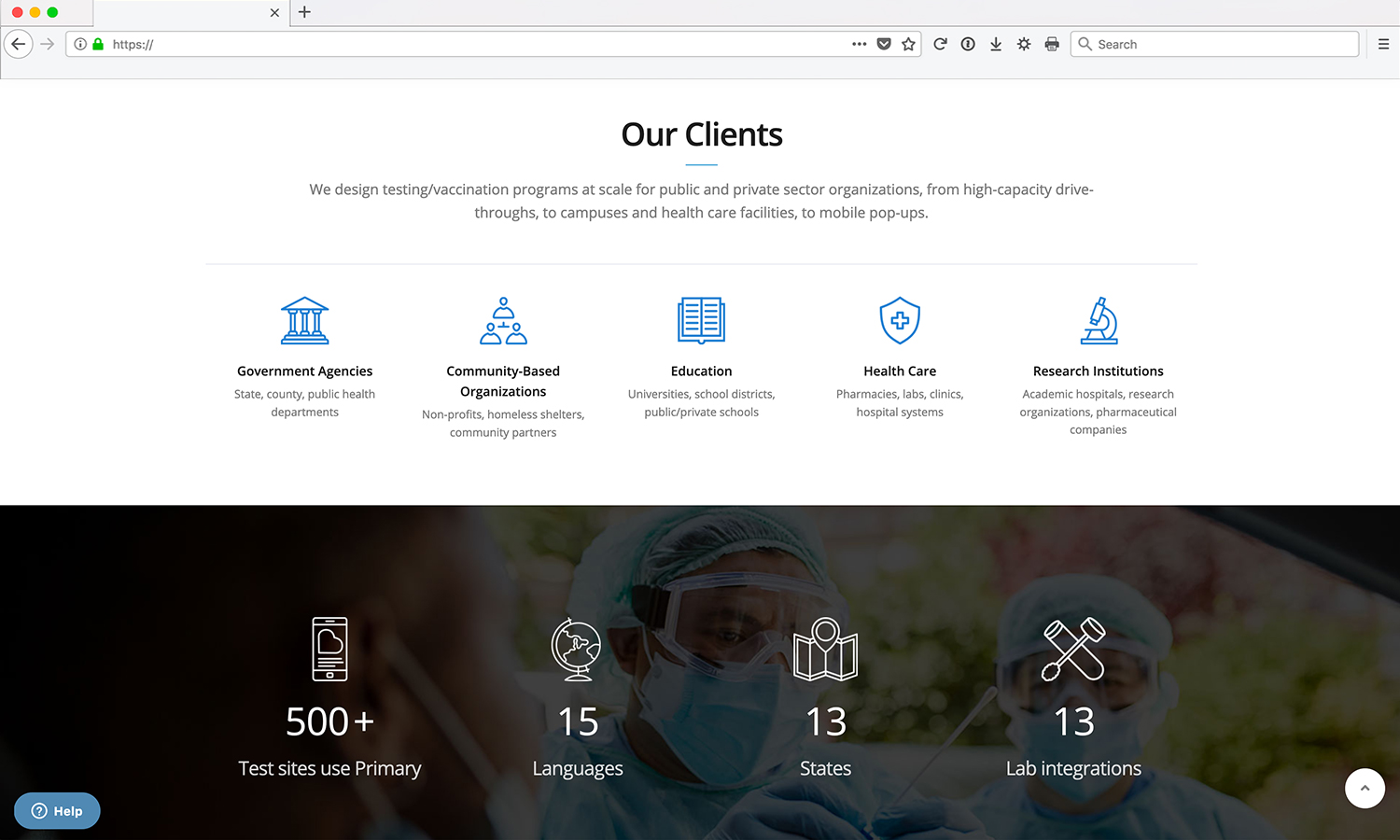In the image, there is a vibrant array of colors and symbols including red, yellow, green, and gray arrows pointing left and right. Letters like H, D, B, and S are prominently displayed along with icons for printers, search tools, and refresh functions. The setting appears to be the Texas Heart Clinic where professionals engage in the design, testing, and assessment of functional programs aimed at both public and private sector positions.

The programs cater to a vast spectrum—ranging from high-capacity drives and expansive healthcare campuses to flexible, mobile pop-up units. The architectural backdrop includes various buildings associated with government agencies at the state and county levels, public health departments, community-based organizations, non-profits, homeless shelters, and community partners.

Education is also well-represented, with mentions of universities, school districts, and both public and private schools, indicated by an open book icon. Healthcare organizations form another core component, encompassing pharmacies, laboratories, clinics, hospital systems, academic hospitals, research organizations, and pharmaceutical companies, depicted by a microscope.

Toward the bottom left corner, three blue symbols signify health and testing sites, suggesting that primary services are provided in as many as 15 different languages, depicted by a globe icon. Additionally, there are 13 laboratory integrations and a person appears in the background, emphasizing a personal or human aspect. The image is dense with information, symbolizing a comprehensive approach to health, education, and community welfare services.